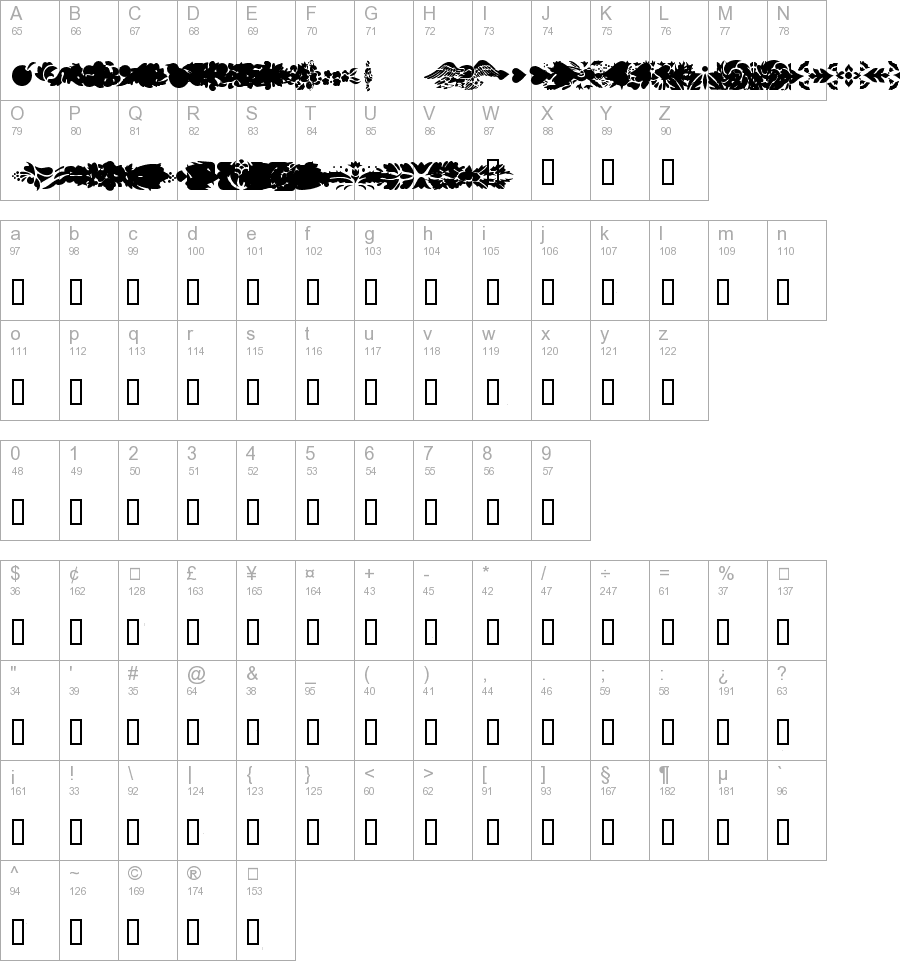The image features a comprehensive character set displayed against a white background. This set includes a sequential list of characters starting with uppercase alphabets from A to Z, followed by lowercase alphabets from a to z. Next, the numeric digits from 0 to 9 are represented. The set also includes a variety of symbols: 

- Monetary symbols: dollars ($) and cents (¢)
- Several punctuation and typographical symbols: a plus sign (+), minus sign (-), asterisk (*), forward slash (/), percent sign (%), at symbol (@), ampersand (&), underscore (_), period (.), comma (,), semicolon (;), colon (:), exclamation mark (!), and question mark (?)
- Other symbols: inches and feet denoted by double quotes (") and single quotes ('), respectively, as well as an upside-down question mark (¿)
- Mathematical and logical operators: equal sign (=) and vertical bar (|)
- Parentheses and brackets: left parenthesis ((), right parenthesis ()), left bracket ([), and right bracket (])
- A variety of other symbols: pound (£), yen (¥), and a backslash (\).

Each character and symbol is distinctly displayed for clear identification.